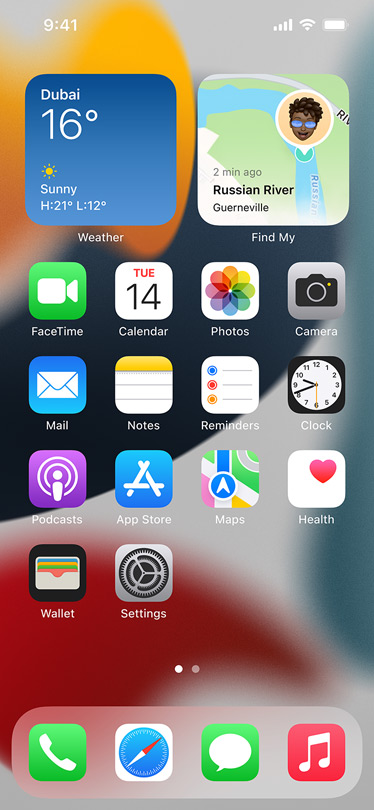This is a screenshot of a mobile phone’s home page with an abstract, blurred background featuring various colored shapes. In the upper left corner, there’s an orange shape, centrally located and blending into a dark gray gradient. Below this gradient towards the right is a white shape. At the lower left corner, there is a dark red shape, while on the right side, there’s a grayish-blue shape. 

At the top left, white numerals display the time as "9:41." To the top right, three icons are visible: a set of five mobile signal bars, a Wi-Fi symbol, and a full white battery icon. Below these icons are two large, rounded tiles.

The first tile on the left has a gradient blue background that transitions from darker on top to lighter at the bottom. In the top left of this tile, white text reads "Dubai," followed by "16°" underneath. In the bottom left corner, there is a yellow sun icon, underneath which it reads "Sunny" in white text. Further below, it details the high and low temperatures, "H: 21°, L: 12°." Below this tile, a white label reads "Weather."

The second tile on the right displays a map with green and gray land areas, a curving blue river, and a gray road also at a curve above the river. A teal circle with a white outline is located within the river. Emerging from this teal circle is a white circle connected to it by a small triangle. Inside this white circle is a filled yellow circle featuring a face with blue sunglasses. The tile is titled "Russian River" in black text.